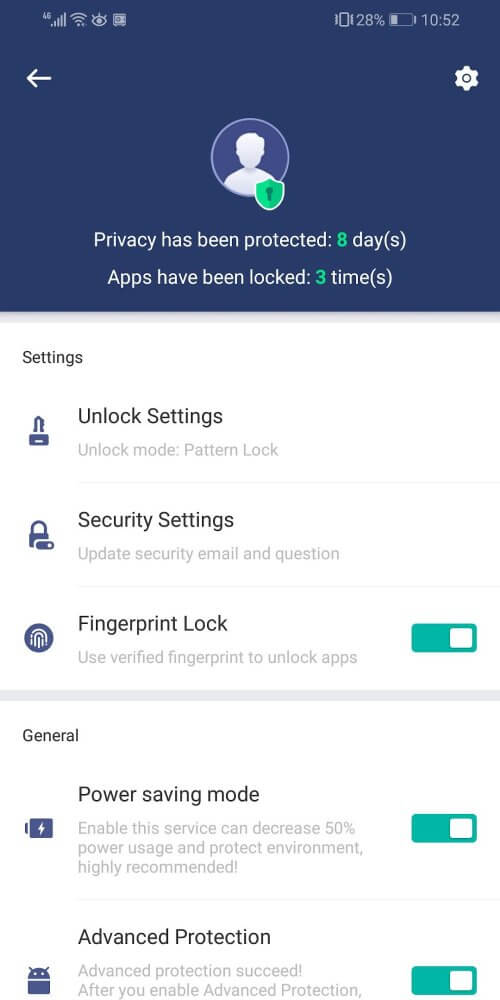A detailed screenshot of a smartphone's settings is displayed, predominantly on a white background with the top third positioned on a blue backdrop. Starting at the top left corner, a service indicator, Wi-Fi symbol, eye icon, and a square shape are visible. On the top right, there is a phone icon, "28%" battery percentage, a battery indicator, and the time, marked as "10:52". Below this, a white back arrow on the left contrasts with a cog icon symbolizing options on the right.

In the blue section below, a profile picture is adorned with a green shield icon beside the text: "Privacy has been protected for eight days, apps have been locked three times." The numbers eight and three are highlighted in white. Transitioning into the white section, there is a series of settings options listed as follows: "Settings," "Unlock Settings," "Security Settings," and "Fingerprint Settings." Each option is accompanied by blue icons: a key, a lock, and a fingerprint. The "Fingerprint Settings" option includes a toggle switch, switched on, indicated by the color green.

A light gray bar divides this area. Below this bar, within another white backdrop, the text "General" appears in black, followed by "Power Saving Mode" and "Advanced Protection," each with toggle switches turned on. Icons next to these options depict a battery for "Power Saving Mode" and the Android logo for "Advanced Protection." Additionally, the image includes various sections of light gray text that are mostly indistinct and not critical to the primary content.